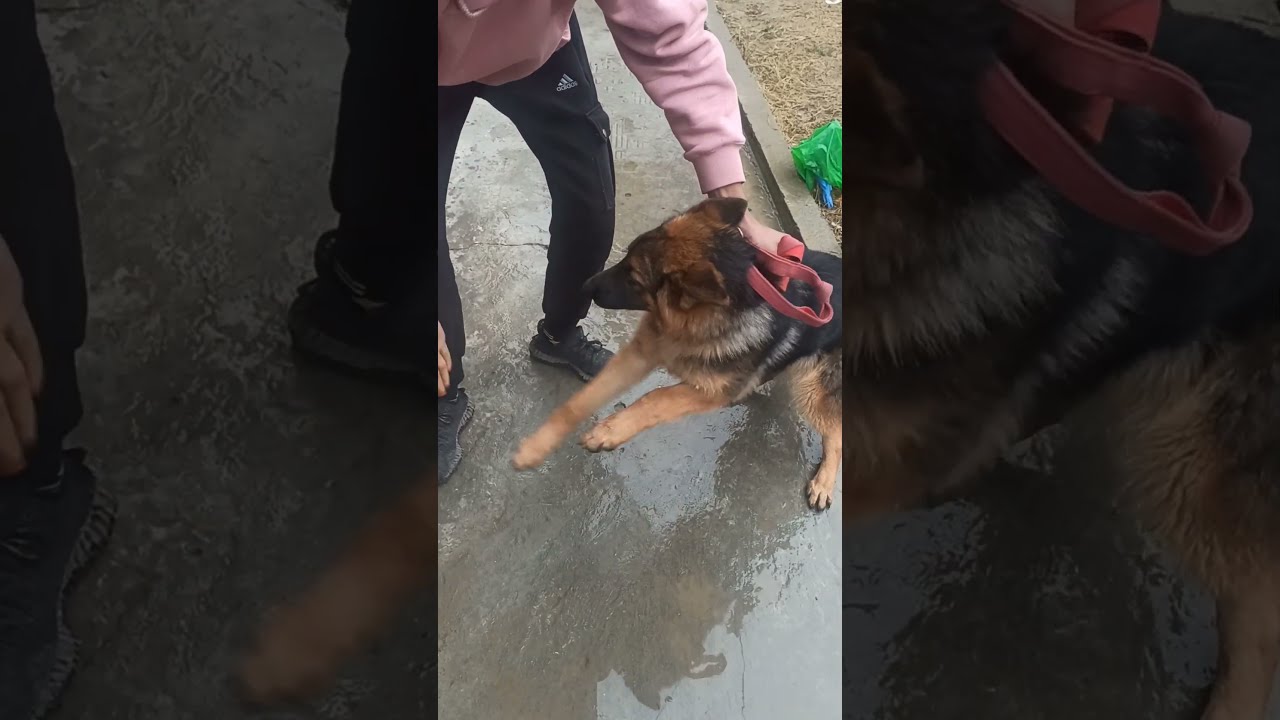The image captures an outdoor scene featuring a gentleman of Caucasian descent, visible from the mid-torso down. He is wearing black pants, black shoes, and a long-sleeve pink or light burgundy sweatshirt. His left hand holds the collar of a German Shepherd, which is restrained by a bundled, light red leash. The dog, characterized by its black fur on the upper body, ears, and muzzle, as well as its darker brown and light tan legs, is up on its hind legs, appearing resistant or uncooperative. They are standing on a wet, reflective concrete surface. The photo also includes two enlarged and darkened zoomed-in sections on either side: one on the left highlights the man's shoes, while the one on the right focuses on a close-up of the German Shepherd.